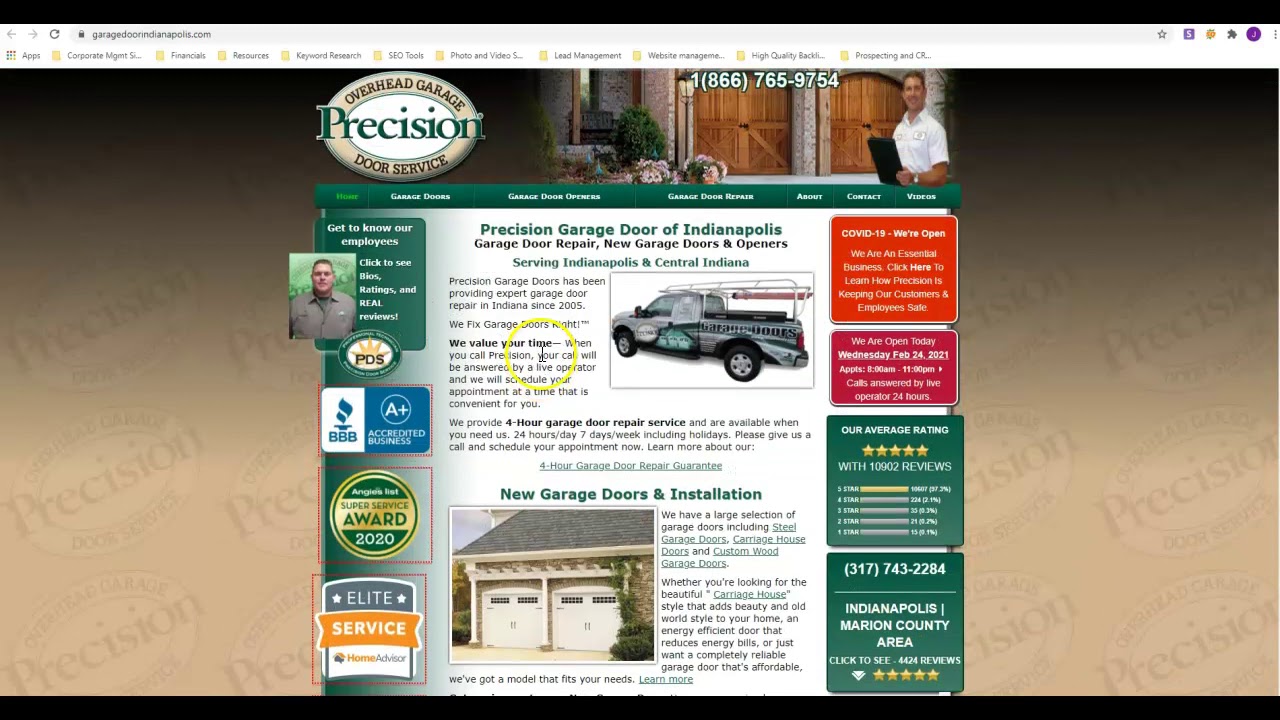The webpage for Precision Overhead Garage Door Service is displayed on a computer screen with a light tan background featuring a watermarked Precision Overhead Garage Door Service emblem. The top and bottom of the page are framed by black banners that stretch horizontally across the screen. 

Dominating the central area of the page is a main content section. At the top of this section, there's a banner showcasing an image of two elegant wooden garage doors resembling those of a carriage house. Standing to the far right of this image is a smiling Caucasian male worker, clad in a short-sleeved white shirt and carrying a black checkerboard. He sports a wristwatch on his left arm, light brown hair, and is positioned against a backdrop of a brick building adorned with shrubs and flowers.

Directly below the image banner is a green rectangular strip with white text listing navigation options: "Home," "Garage Doors," "Garage Door Openers," "Garage Door Repair," "About," "Contact," and "Videos." 

Further down, the page is divided into three sections from left to right: "Get to Know Our Employees," followed by "Click to See Bios," "Ratings and Reel Reviews." Centered on the page is a prominent text block that reads: "Precision Garage Door of Indianapolis," "Garage Door Repair, New Garage Doors, and Openers serving Indianapolis and Central Indiana."

To the far right is an orange square with white text announcing, "COVID-19: We're Open. We're an Essential Business. Click Here to Learn How Precision is Keeping Our Customers and Employees Safe." 

Beneath this announcement is a red rectangle with white text stating, "We're Open Today, Wednesday, February 24th, 2021." Continuing downward, the page displays their average rating and reviews, followed by a contact phone number for visitors seeking services.